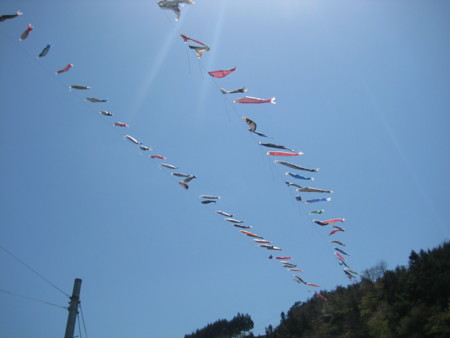The photograph captures a bright blue sky with two prominent sun rays emanating from the middle top of the image, although the sun itself is not visible. Two diagonal lines stretch from the top left corner to the bottom right, adorned with various colored flags or windsocks flapping in the wind. These flags appear in shades of red, blue, green, pink, and black, and differ in sizes and lengths. The lines create an intersecting pattern and terminate in what appears to be a hillside covered in shadowed, overgrown grasses and shrubbery in the bottom right corner. The lower left corner of the image features the top of a utility pole with wires extending from it in various directions. The overall photo has a slightly out-of-focus quality, making some details, such as the exact appearances of the flags and the hill, unclear. This image evokes a sense of an outdoor scene taken from the ground looking up, highlighting the vibrant yet serene atmosphere of a sunlit day.